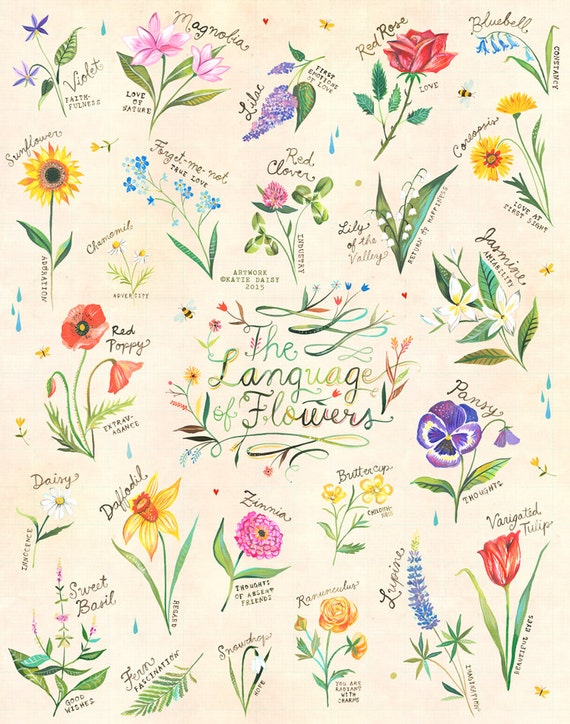The image is a vertically-oriented collage of various meticulously sketched flowers displayed against a beige background, resembling a page from an old botanical journal. At the center, cursive text reads "The Language of Flowers," with each letter in shifting hues of green, yellow, and brown. The drawings, seemingly done in colored pencils, feature a vibrant array of colors such as purple, pink, red, yellow, orange, blue, peach, and lilac, enriched with shades of white. 

Each flower is labeled in cursive and accompanied by a word or phrase denoting its symbolic meaning. Starting from the top, notable flowers included are a violet symbolizing faithfulness, a magnolia representing the love of nature, a lilac denoting the first emotions of love, a red rose symbolizing love, a bluebell for constancy, a sunflower representing addiction, chamomile with its tiny white petals and yellow center (though the corresponding word is unreadable), forget-me-nots indicating true love, and a red clover standing for industry. The meticulous details and diverse hues make the piece both visually appealing and rich in symbolic significance.